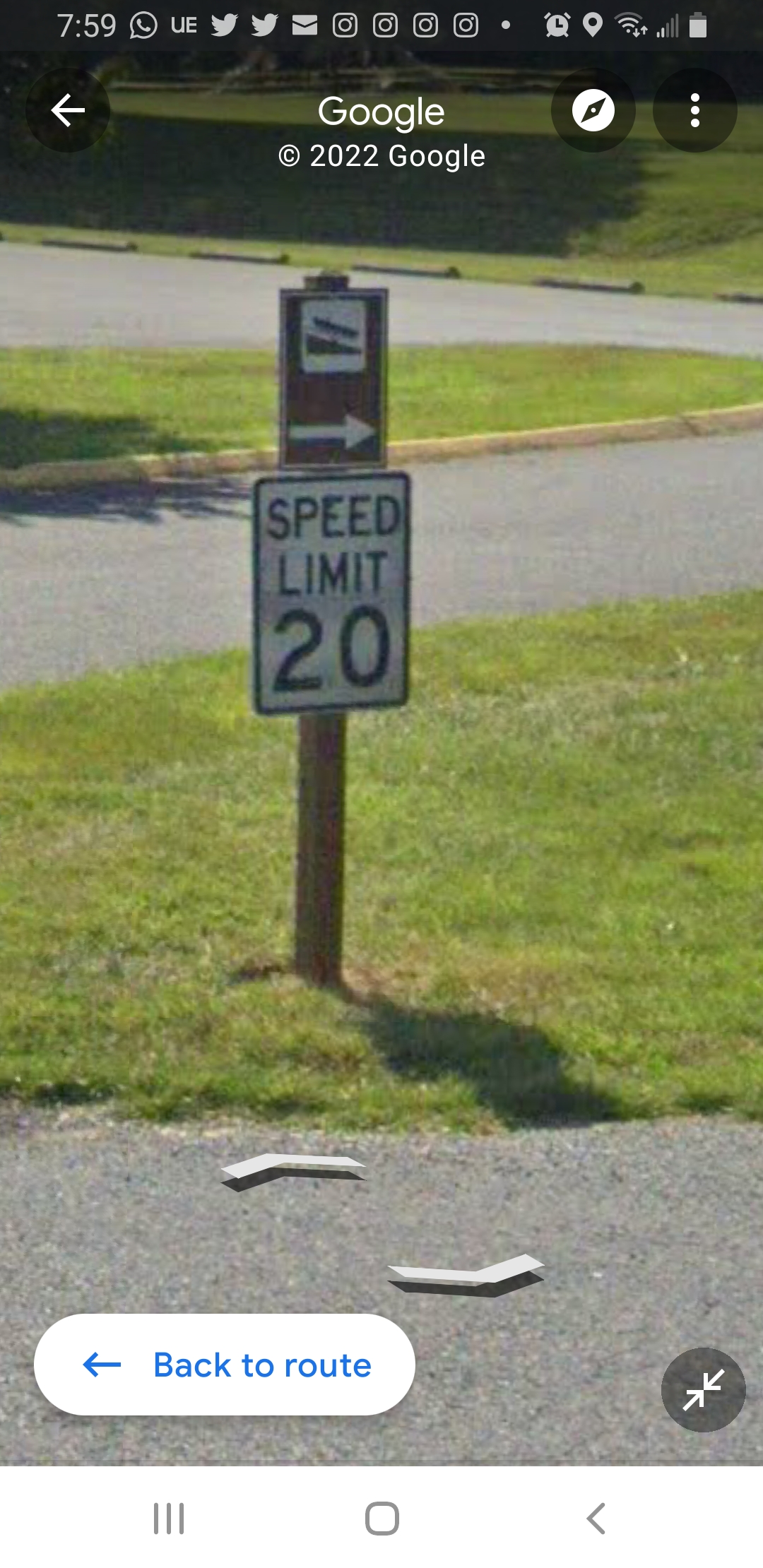A detailed Google Street View image captures a scene in what appears to be a park or recreational area, characterized by the absence of sidewalks, indicating it's likely part of a parking lot. The focal point of the image is a speed limit sign, conspicuously shorter than average, standing approximately five feet tall. Situated atop a sturdy wooden post, this utilitarian sign integrates with the surrounding patch of grass, contributing to the park-like aesthetics.

Above the speed limit sign, another brown sign with a directional arrow pointing to the right is mounted. Although there is an image on this brown sign, its specifics are indistinguishable. The background reveals another road and an additional parking lot, further reinforcing the functional landscape. The implicit tranquility of the grassy area suggests a well-maintained environment typical of public parks.

The image is a screenshot from a phone, capturing an array of digital notifications and indicators overlaying the top. These include Instagram and Twitter notifications, the current time, battery life, GPS status, and an alarm icon. At the bottom, the image is stamped with a "2022 Google" copyright notice, alongside navigational options such as "Back to route" and a GPS indicator, hinting that the screenshot was taken during an active navigation session using Google Maps.